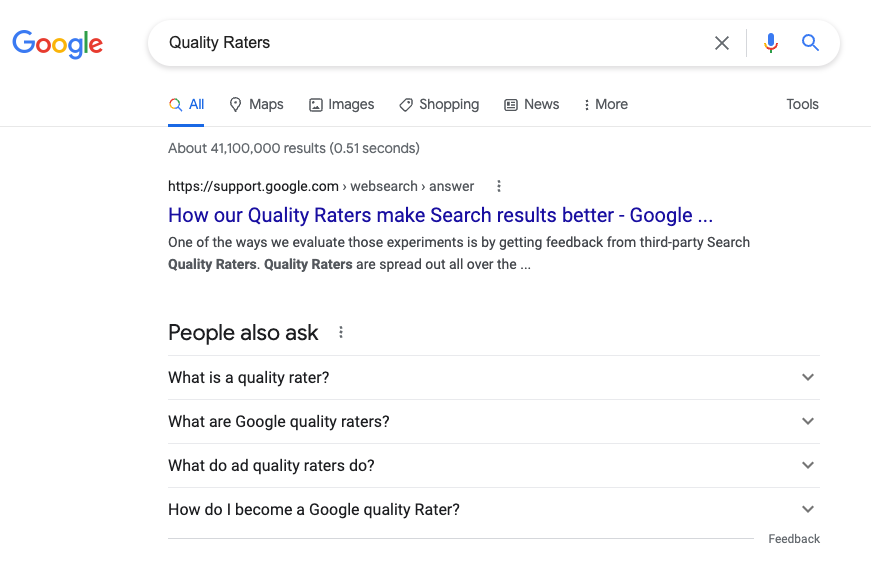A detailed screenshot of a Google search results page. The Google logo is prominently displayed on the left side of the search bar, which contains the query "quality Raiders." Icons for clearing the text, voice search, and executing the search are also visible within the search bar. Below this is a navigation menu listing categories like All, Maps, Images, Shopping, News, More, and Tools positioned to the far right.

In gray text, it indicates there are approximately 41,000 results generated in 0.51 seconds. The first search result begins with a website header in black text followed by a link in blue text that reads "How Our Quality Raters Make Search Results Better - Google." Below this, black text describes the content briefly: "One of the ways we evaluate those experiments is by getting feedback from third-party search quality raters. Quality raters are spread out all over the..."

Following this, the "People also ask" section appears in bold black text, featuring a gray dropdown bar. It includes expandable questions such as "What is a quality rater?" "What are Google quality raters?" "What do ad quality raters do?" and "How do I become a Google quality rater?" To the right of this section, there's a "Feedback" button. The remainder of the screenshot provides no additional information.